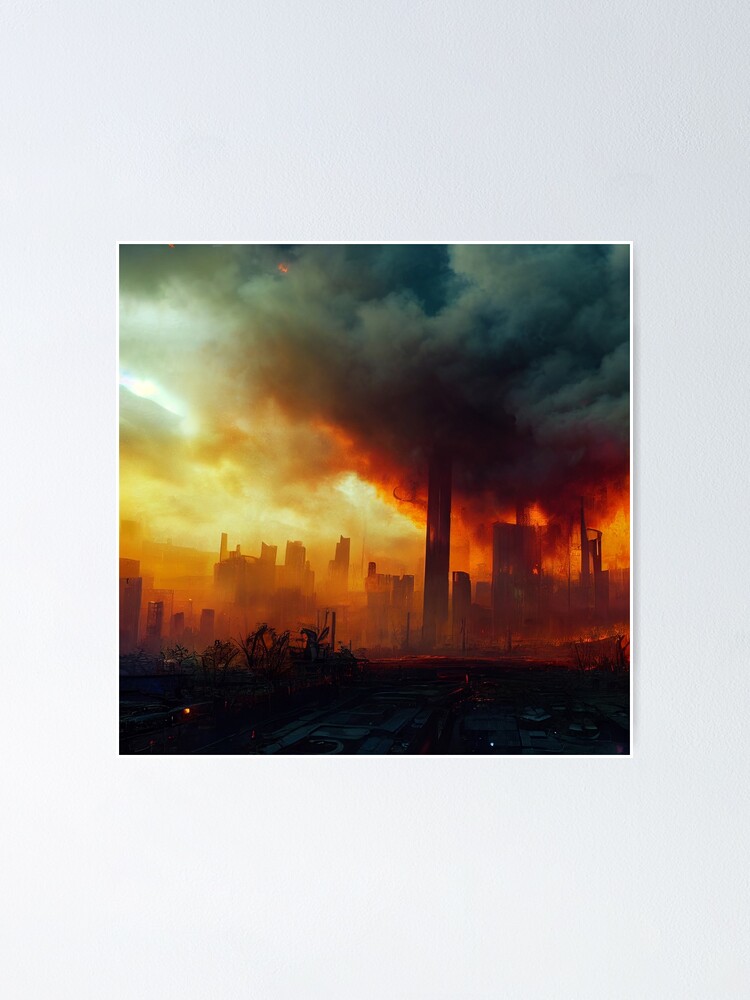The photograph, framed with a very thin white border, depicts a post-apocalyptic cityscape viewed from a vantage point that suggests standing on a dark, shadowy hill, perhaps in a park or an abandoned lot with sparse, struggling plant life. The foreground is overwhelmingly dark, almost black, with hints of shrubs. Central to the image is a city engulfed in ominous, gray smoke emanating from a massive plume in the upper right corner, which sharply contrasts against the ethereal light gray wall in the background. The city's tall structures are partially silhouetted by a fiery orange and yellow sky, suggesting an ongoing disaster, likely a massive fire. The left side of the sky has a golden haze, hinting at pollution, while the entire urban scene bathes in a polluted, apocalyptic glow. In the far distance, the silhouetted hills contribute to the unsettling, desolate atmosphere.